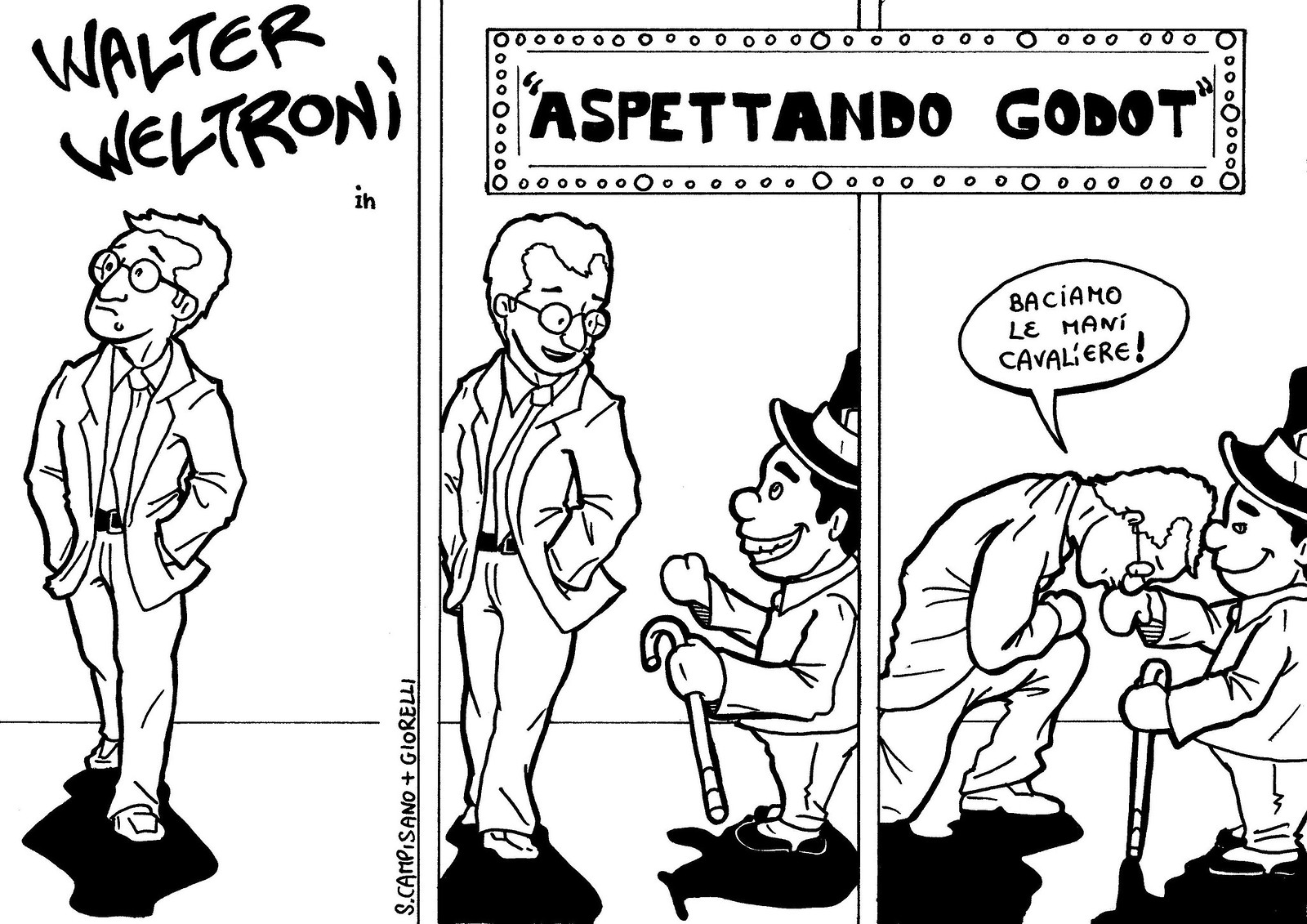This black and white comic strip is divided into three panels. The first panel features a text in bold font that reads "Walter Weltron, Weltroni," above a bespectacled, suit-clad man who resembles Woody Allen, standing in a room with his hands in his pockets, gazing upwards towards his left. There's a prominent shadow beneath his feet. In the second panel, atop the scene, is a Broadway-style marquee sign with lit-up circles around it, displaying the title "Aspantando Gudo." Below, the same man is now looking at a much shorter, elf-like figure wearing a top hat and holding a cane. The third panel shows the taller man kneeling and kissing the hand of the shorter, leprechaun-like character, with an exclamation-filled speech bubble above him reading "Basiamo le ho calviliere!" or a similar phrase, indicating an exuberant expression in a possibly Spanish or Italian language.